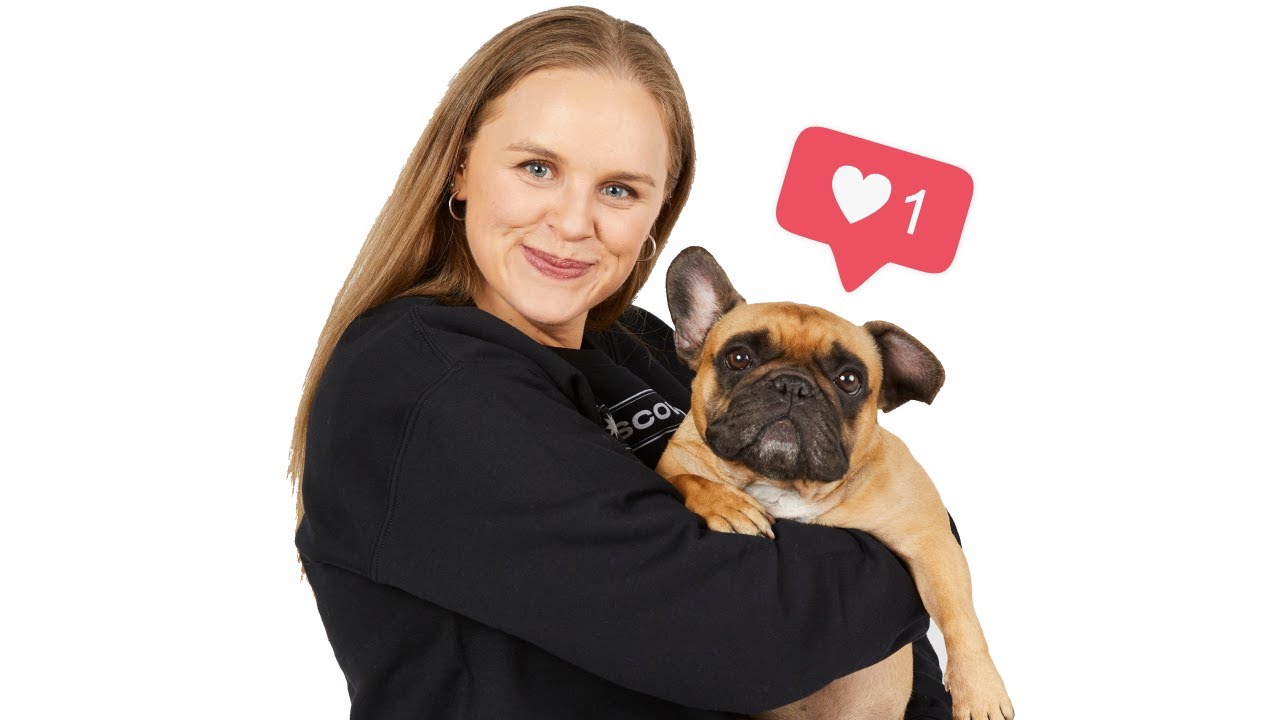This digitally-enhanced, full-color promotional image depicts a horizontally rectangular scene with no border, set against a grayish background. The image is centered around a striking dog, likely a beagle, whose unique features capture immediate attention. This beagle, with its orangish-brown and white coat, is adorned in a white shirt and a black collar. Particularly notable are its heterochromatic eyes—one light blue and the other a yellowish-brown. 

The beagle stands prominently on the left half of the image, facing the camera. The dog's coat includes a white snout and forehead, with a distinct white strip running down the center of its head. The sides of its face and eye area exhibit a light brown shade, blending into an orangish hue on its neck.

Adding to the visual intrigue are artificial sunspot-like lighting effects: a green light on the left casts a slight green tint on part of the beagle's face, while two white lights on the upper right, one large and one small, resemble stage lights. 

Text positioned along the center-right reads "Dog Fashion Show" in bold, light green lettering with a darker green shadow, giving it a three-dimensional appearance. The overall composition creates a dynamic and eye-catching promotional piece for a dog fashion show.